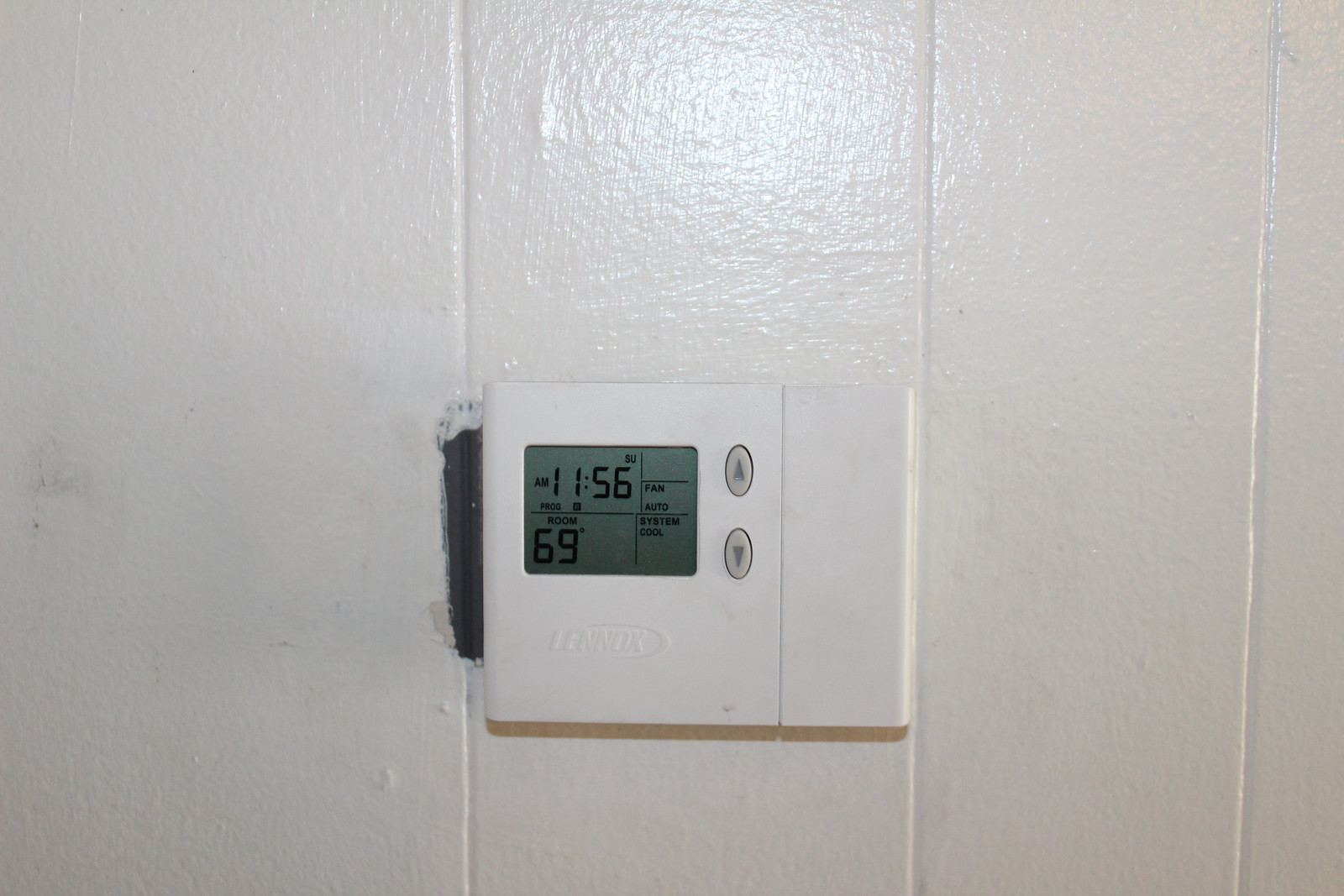The image features a white Lenox thermostat affixed to a wooden wall, painted white. The digital display on the thermostat shows the current time as 11:56 a.m. on a Sunday and indicates that the room temperature is 69 degrees Fahrenheit. Below the display, there are options for "Fan," set to "Auto," and "System," set to "Cool." The thermostat is equipped with up and down arrow buttons, presumably for adjusting the room temperature and making various selections. 

The wooden wall to which the thermostat is mounted exhibits visible lines and texture, and there appears to be some peeling around the area where the device is attached, possibly due to age or installation wear. The overall color scheme is monochromatic, with the white of the wall and thermostat blending together, contrasted only by the gray buttons and screen on the thermostat.